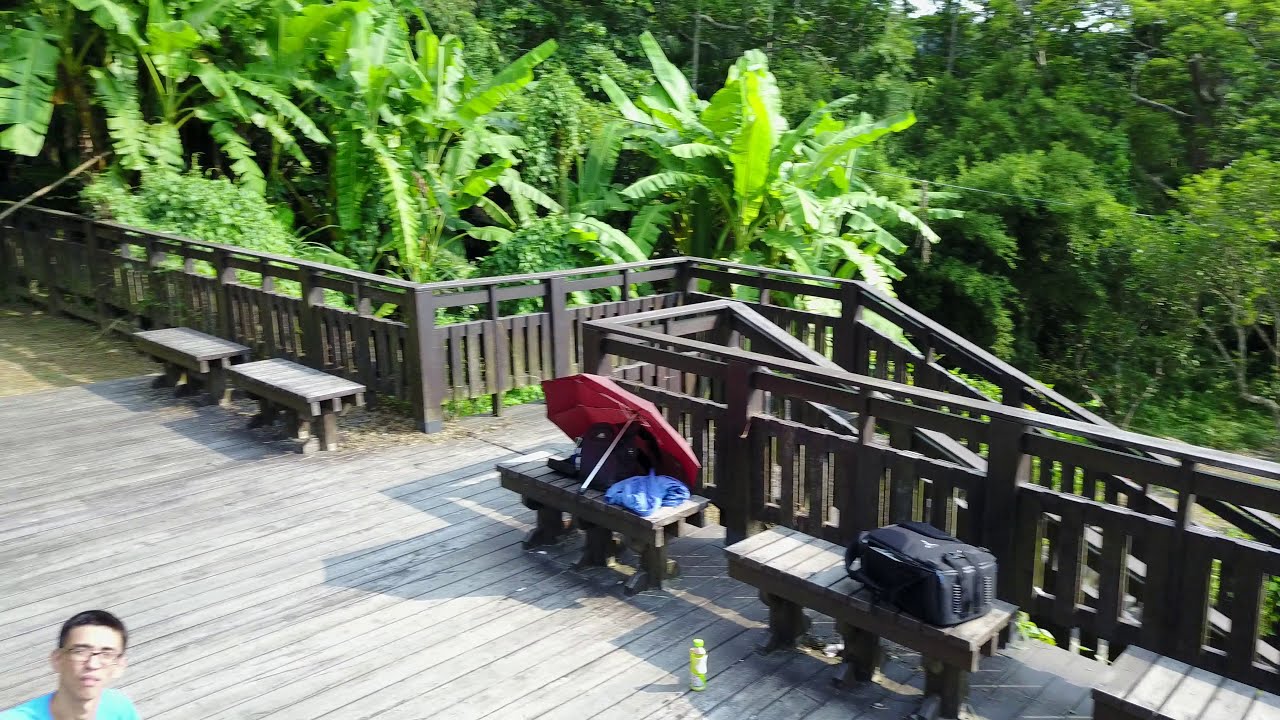The image depicts a large wooden deck extending from the upper left corner to the bottom right corner, furnished with five small benches. The deck has a brown wooden railing that runs diagonally, leading to a set of stairs descending from the middle of the deck. Two of the benches, located in the lower part of the image, have a black bag and a red umbrella with another black bag respectively. A small figurine is placed on the deck floor in front of these benches. In the background beyond the railing, a dense wooded area filled with light and dark green trees and bushes can be seen. In the bottom left corner, there is a man with glasses, short black hair, and a light blue shirt, visible from the shoulders up.